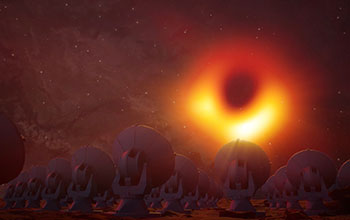This detailed image captures a surreal and otherworldly landscape, primarily characterized by a night sky that's both dark and intricately wrinkled, filled with a dense scattering of stars that set it apart from Earth's familiar nightly view. Dominating this alien sky is a vibrant, donut-shaped orange light with a black center, reminiscent of an eclipse, shedding bright illumination over an entire scene. The ground before us reveals a multitude of identical, round radio dishes or satellite-like structures, each equipped with a base and an anchor, all perfectly synchronized and oriented towards the bright orange object in the sky. These structures stretch endlessly in rows to the left, right, and into the distance, reflecting hues of red and orange, as if bathed in the luminous glow of the celestial phenomenon above.